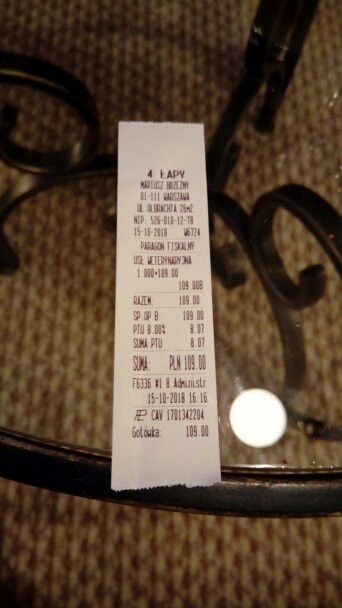A photograph captures a long, foreign-language receipt placed atop a transparent glass coffee table. The receipt details a purchase totaling 109 units of an unidentified currency, approximating $100 worth of products. The glass table is highly transparent, offering a glimpse of the carpet below and creating a subtle reflection of the receipt. The table features a sleek, metallic rim and an intricate design with three legs converging at the center, visible through the glass surface.